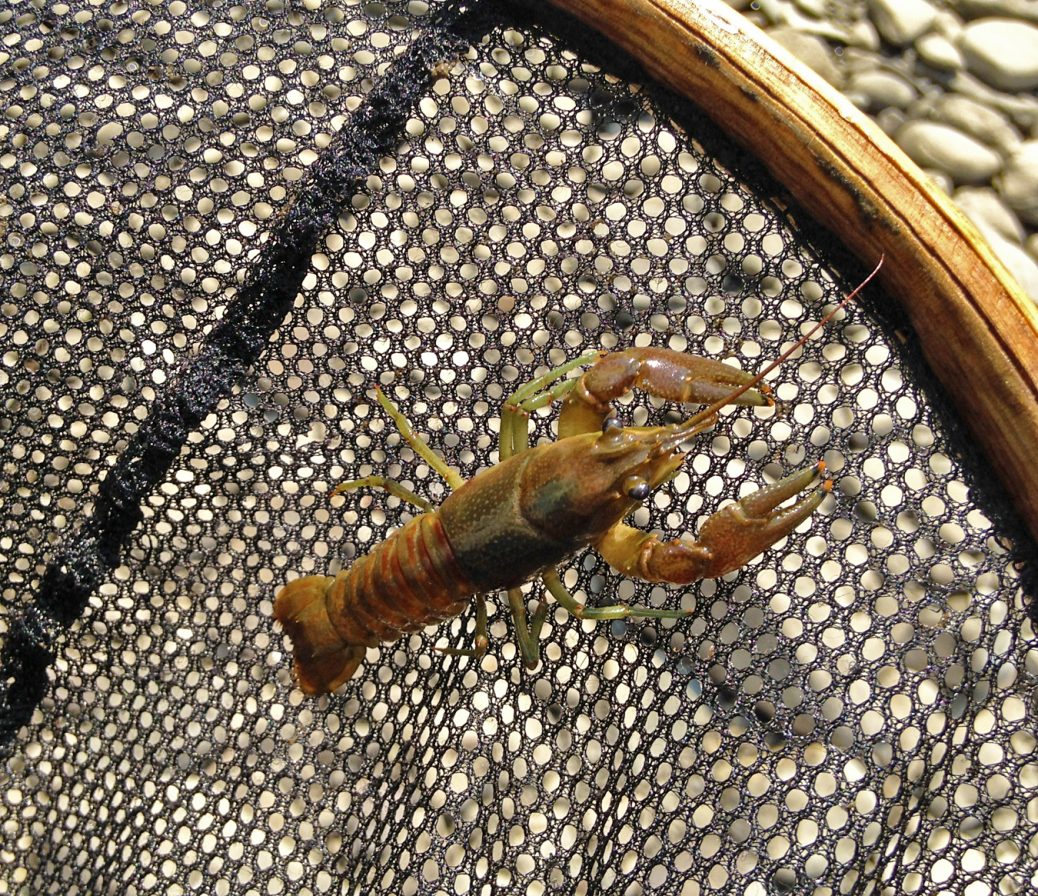A detailed close-up image features a small lobster striving to escape a black fishing net with a wooden rim that circles its perimeter. The lobster, which exhibits a range of pale reddish to brown hues characteristic of a live specimen, is the focal point of the image. Its distinct body parts include long tentacles extending from its head, brown pinchers, and multiple smaller legs tinged with shades of green. The creature's effort to climb up the net suggests it aims to return to the blurred, rocky shoreline visible in the background. This shoreline, likely situated near water, stretches out of focus, emphasizing the lobster's struggle and highlighting the intricate details of its form.